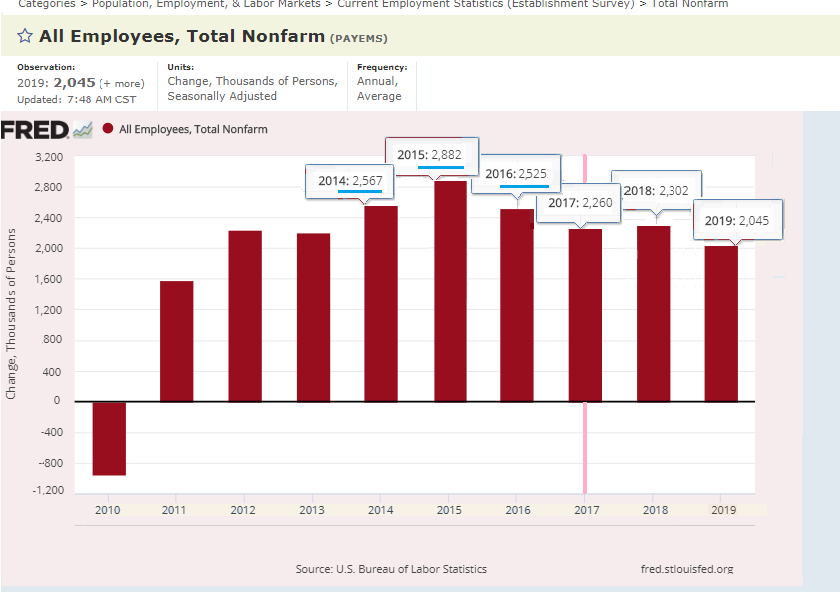The image is a detailed data visualization in the form of a vertical bar chart, possibly a screenshot from a web page, given the presence of a breadcrumb trail at the top. The breadcrumb reads, “Categories > Population, Employment, and Labor Markets > Current Employment Statistics > Establishment Survey > Total Non-Farm,” indicating the hierarchical navigation. 

The title of the chart in black on a cream background states, "All Employees: Total Non-Farm (PAYEMS)." The chart includes sections for observation units, frequency, and a logo labeled "FRED." A maroon circle in the legend specifies "All Employees: Total Non-Farm."

The x-axis displays years from 2010 to 2019, while the y-axis measures changes in thousands of persons, starting at zero and ranging from -1,200 to 3,200. Each bar represents annual data: the year 2010 shows a negative value of approximately -900, and from 2011 onwards, all values are positive, with the highest being around 1,600 in 2011. Bars from 2014 to 2019 have specific values noted, likely from mouse-over details, including values like 2,567. At the bottom, the source is cited as the U.S. Bureau of Labor Statistics, and the site is identified as fred.stlouisfed.org.

The background of the chart is white, with a yellow stripe across the top where the main title is found. The chart background switches to pink beneath the header to highlight the bar chart area. The chart effectively visualizes the changes in the total non-farm employment over a decade, clearly displaying the transition from negative growth in 2010 to consistent positive growth in subsequent years.